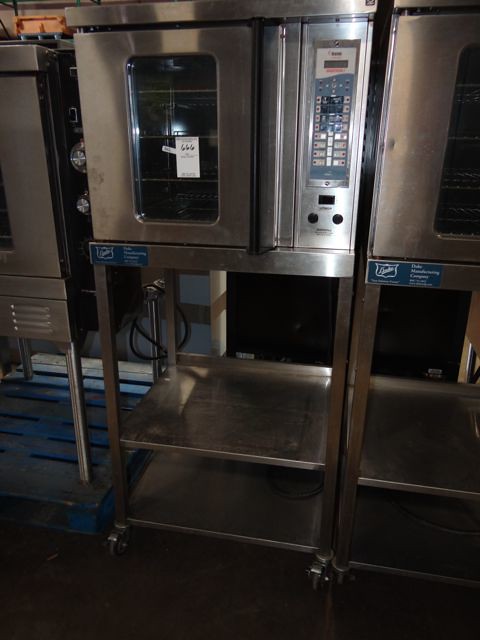The photograph captures a well-lit industrial kitchen scene focused on a stainless steel piece of equipment that resembles an oversized microwave or proofer. This central appliance, positioned on a stainless steel rolling stand, features two lower shelves—a smaller one at the bottom and a second midway up—with a significant gap between the top shelf and the main body of the machine. The upper part has a clear window revealing internal racks and a control panel with several push buttons on the right-hand side. The equipment, potentially used in commercial cooking or baking settings, is flanked by similar stainless steel appliances, with one possibly having a blue pallet-like base. A visible sticker on the glass of the central unit hints at pricing, though the details are obscured except for a partial figure '666'. The floor is largely obscured but appears to have a bluish tint in the background, with the wall's color remaining indeterminate due to poor lighting.